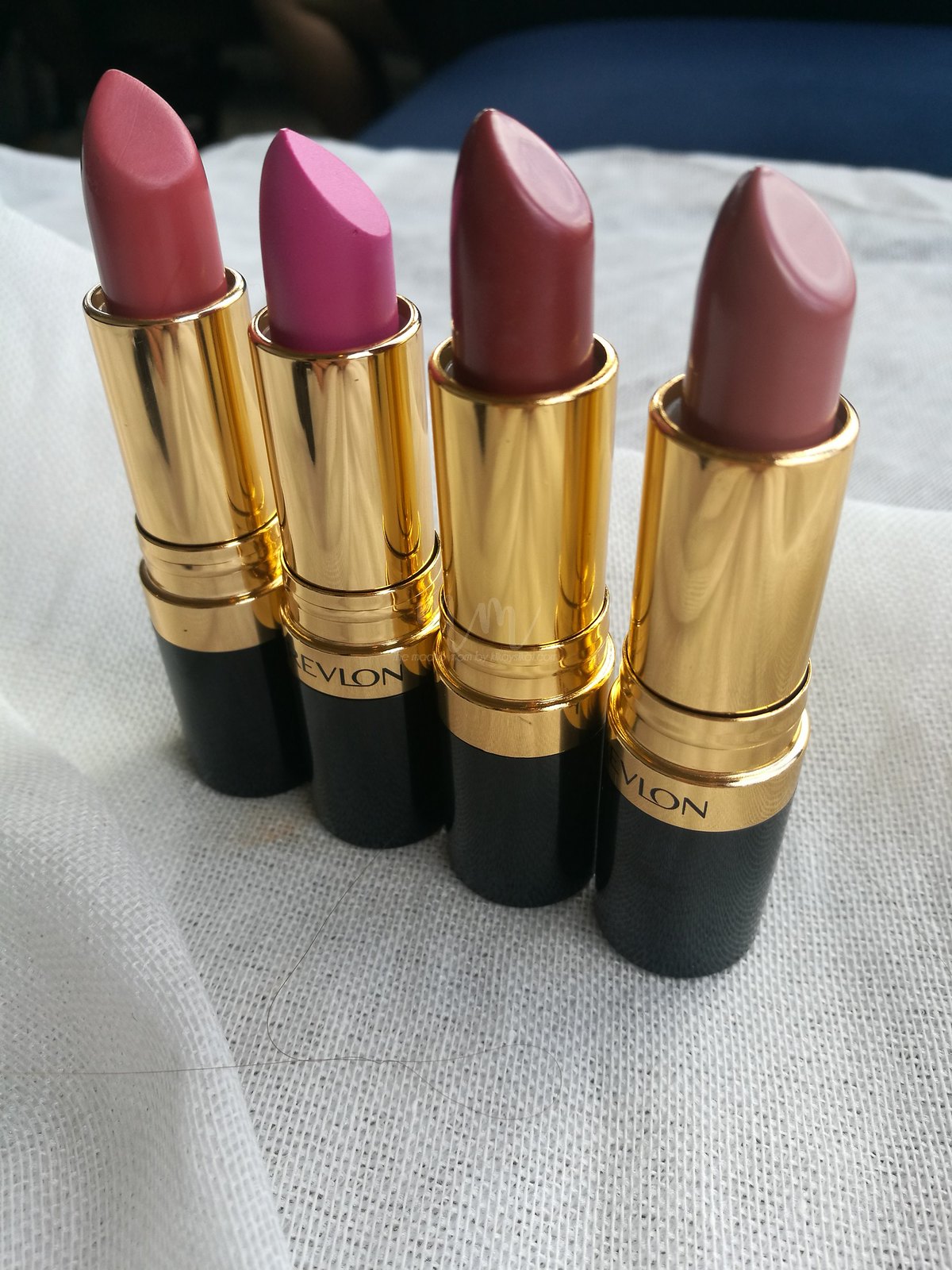This color photograph, bathed in natural light offering a soft and inviting tone, features four Revlon lipsticks standing upright in a diagonal line from the center left to the bottom right. Each lipstick is open and twisted up, revealing their pristine and fresh condition. They sit on a white mesh fabric, which adds texture and contrast to the scene. The lipsticks, adorned with shiny gold metal bodies and black bases that have been removed and reattached to the opposite ends, reflect ambient light beautifully. The colors of the lipsticks range from a brownish red, possibly termed Blood Earth, to a pink, a deep rich brown with a hint of red, and a softer caramel brown. The background behind the lipsticks is a blue, indistinguishable blur, adding a serene backdrop to the composition. Notably, the second and fourth lipsticks are branded with the Revlon name, adding a touch of elegance to the overall presentation.